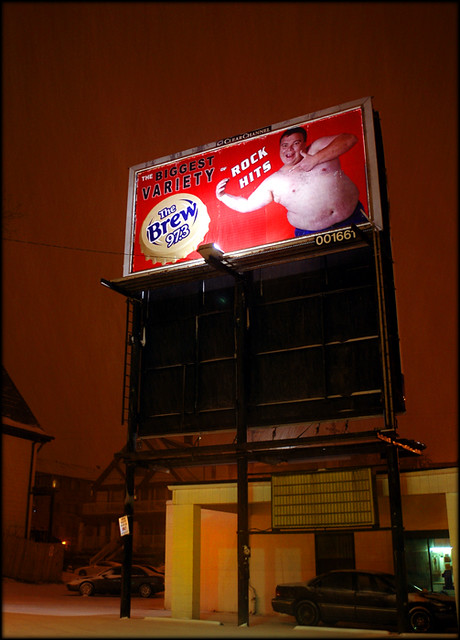This nighttime photograph captures a billboard towering on a tall black metal platform in a modest residential neighborhood. The billboard's red background prominently features a heavyset, shirtless white man, merrily gesturing with his hands. At the top left, within a white bottle cap edged in blue, the logo reads "The Brew 97.3," indicating it's an advertisement for a radio station. The tagline "Rock Hits" appears in bold white letters, followed by the phrase "Biggest Variety" in black below. 

In the background, a second billboard is partially visible, positioned lower and oriented in the opposite direction, though only its backside is seen. Directly below the billboard is a small, one-story building, adjacent to a parking lot with several cars parked both underneath the billboard and around the corner. This scene captures the blend of urban advertising amid a community setting.